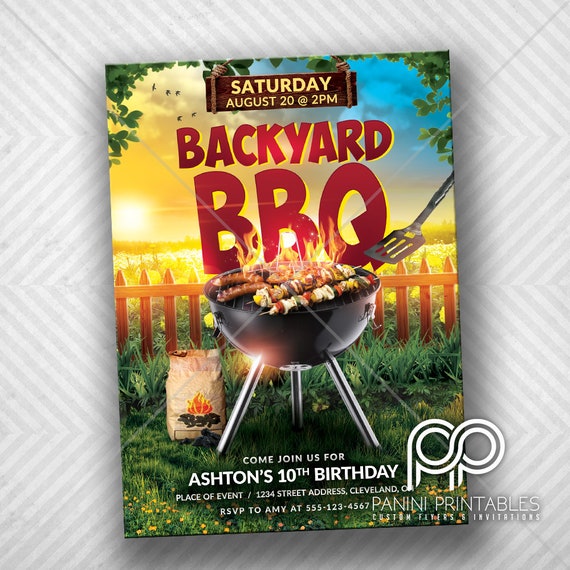The image is a square-shaped birthday invitation with a light gray background featuring a pattern of gray and dark gray stripes and squares. In the center, there is a digitally rendered flyer for a backyard barbecue. The flyer prominently displays a wooden sign in yellow font that reads, "Saturday, August 20th at 2 p.m." Below this, in red font, it says, "Backyard Barbecue." The focal point of the flyer is a cartoon-style illustration of a grill loaded with kebabs and sausages, depicted with flames atop a charcoal barbecue, set on green grass next to a brown picket fence. The backdrop includes a sunrise and a few trees, giving it a welcoming outdoor vibe. The bottom part of the flyer states in white font, "Come join us for Ashton Stanton's 10th birthday," along with the event location, "1234 Street Address, Cleveland, Ohio," and the RSVP contact, "Amy at 555-123-4567." The lower right corner of the image features a watermark in white font that reads, "PP Panini Printables, Custom Flyers and Invitations." This setup demonstrates the type of custom flyer Panini Printables can create for events like a backyard barbecue.